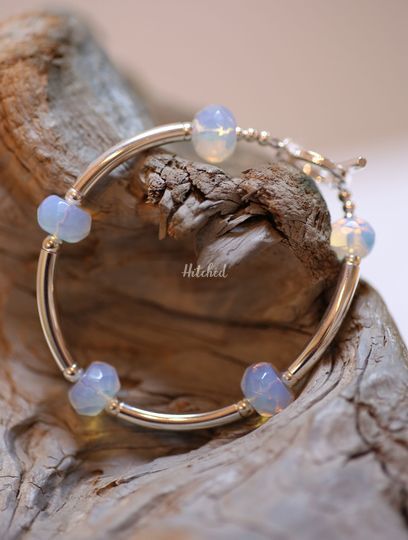This image depicts a small, round bracelet made of a light-colored metal, possibly a golden brass or silver. The bracelet features a clasp along its perimeter and is adorned with five translucent beads, each slightly tinged with blue. The bracelet is presented on a piece of intricately detailed driftwood, centrally located in the photo, though the wood becomes blurred at the top of the frame. The background of the image is a soft, cream-beige color, but it's indistinct and does not provide any additional context. The overall emphasis is on the delicate bracelet and its elegant display.